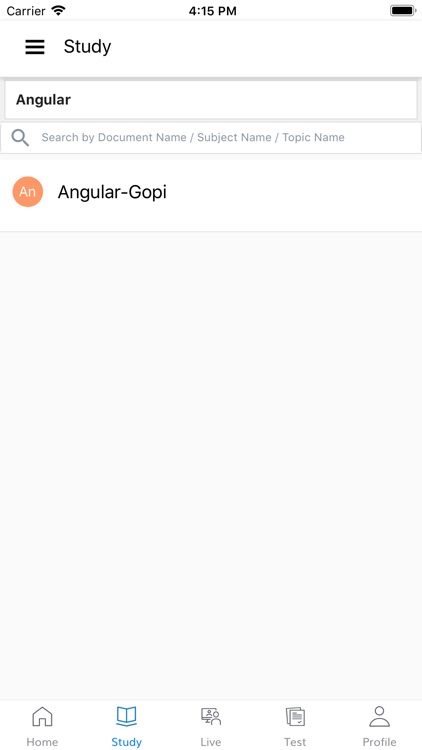This detailed and informative caption describes the user interface of a mobile phone app as captured in a screenshot. 

---

The screenshot displays the interface of a mobile phone app. In the upper left corner, "Carrier" is displayed against a white background with black text, alongside an icon indicating strong connectivity. Centered at the top is the current time, "4:15 PM." On the upper right, a full battery icon is present. 

Below the status bar, there's a section titled "Study," accompanied by three horizontal bars indicating a menu or options. Beneath this header, the text "Angular" appears prominently. Additionally, there is a search field displaying placeholder text, "Search by document name, subject name, topic name." 

An orange circle with the initials "AN" in white is positioned below the search bar, labeled "Angular-Gopi." The main portion of the screen is dominated by a large light gray square, which is empty.

At the bottom of the screen, there is a navigation bar with five icons labeled "Home," "Study," "Live," "Test," and "Profile." The "Study" icon is highlighted in blue and depicts an open book, while the other icons are gray.

---

This refined caption offers a clear and comprehensive description of the screenshot's content.